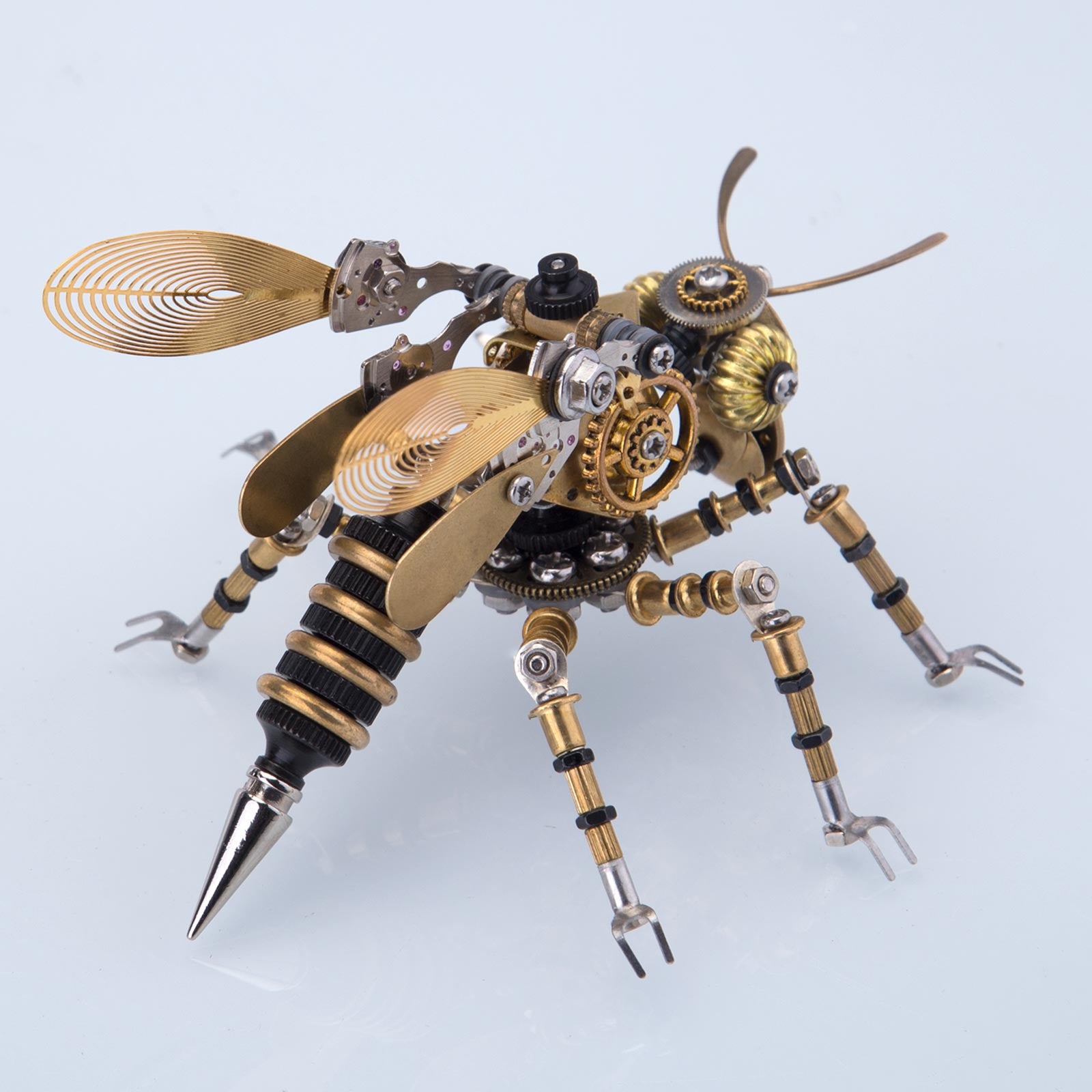In the image, we see a highly detailed mechanical bumblebee rendered in a steampunk fashion. The bee is crafted from an assortment of metal parts, including screws, sprockets, gears, and little metal prongs. Its body showcases a variety of metallic hues such as gold, silver, brass, bronze, and copper. The wings, numbering four, are a gold color and resemble delicate, intricate metalwork, contributing to the bee’s mechanical aesthetic. The stinger, a prominent feature pointing towards the bottom left of the image, resembles a pen point or the top of a wine stopper, emphasizing its sharpness. The legs, six in total, extend from either side of the bee’s body and appear to be made of gold tubes, reflecting the meticulous assembly of found metal objects. The eyes are golden and connected with screws, adding to the robotic appearance. The bee is oriented towards the upper right against a light blue background, highlighting its elaborate construction and the artistic combination of steampunk elements. The overall effect is a striking, gold-eyed, mechanical bumblebee that looks both intricate and plausible in its craftsmanship.